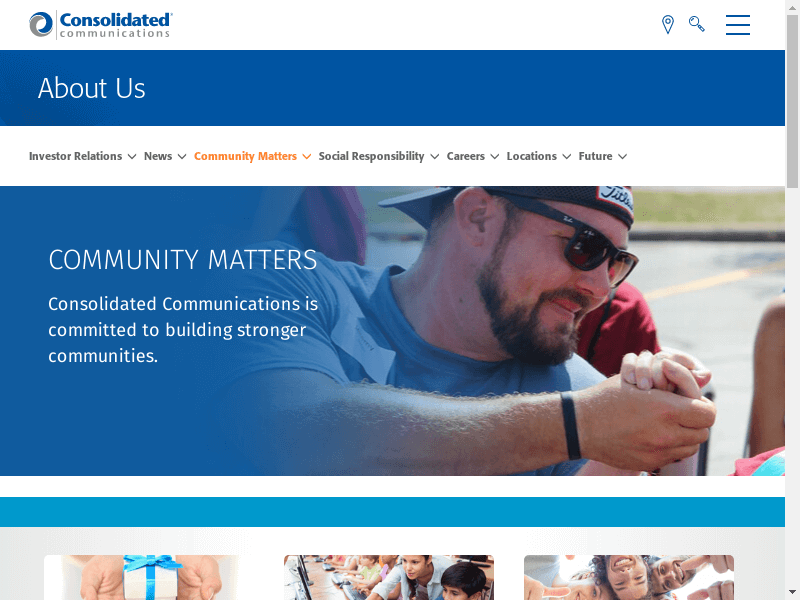This image showcases a website for Consolidated Communications. At the top left corner, the company name "Consolidated" is displayed alongside its logo, which features gray and blue swirls forming a circle. On the top right corner, there are a pin icon, a magnifying glass icon, and a three-line navigation menu icon.

Below the header, there's a blue banner with the text "About Us." Underneath, a white navigation bar features several dropdown options, each marked with an arrow to the right. The options are: "Investor Relations," "News," "Community Matters" (highlighted in orange), "Social Responsibility," "Careers," "Locations," and "Future."

The main section of the page shows a large image of a man with a dark brown beard, wearing a backward hat, glasses, and a blue shirt. He's holding the hand of a child. The text on the image reads "Community Matters" in large white letters and "Consolidated Communications is committed to building stronger communities."

Separated by a white line but highlighted with a thick blue line at the top, the next section displays three partially cut-off images: a pair of hands holding a white and blue present, a group of people using keyboards, and individuals looking down at the camera and giving a thumbs up.